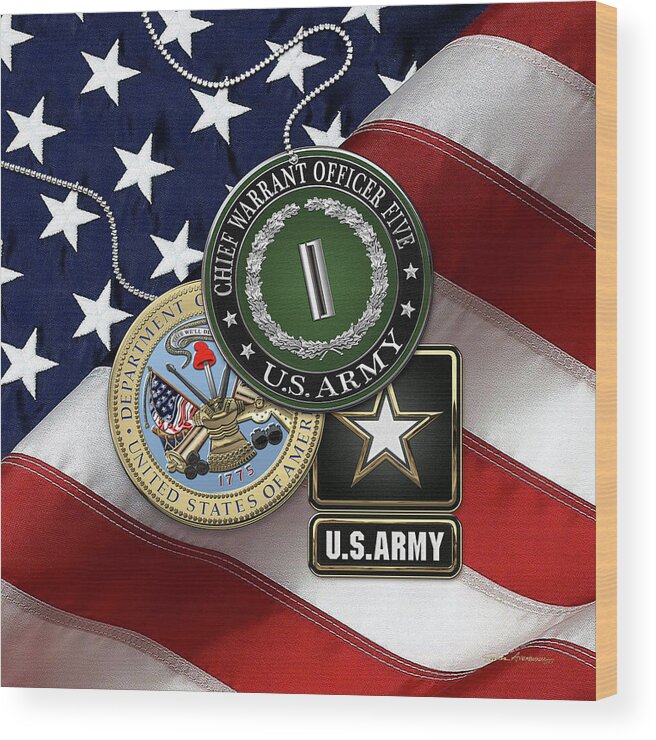This detailed color photograph captures an intricate display centered on a fragment of the American flag, prominently showing the blue field with white stars in the upper left and red and white stripes flowing towards the lower right. The image seems to be mounted on a wooden plaque or within a tiny wooden box, hinting at a commemorative purpose. Central to the composition are three distinct emblems, suspended by a dog chain descending from the upper left corner. The topmost emblem is a green circular patch with black trimming, labeled "Chief Warrant Officer 5 U.S. Army," featuring a single gray bar encircled by a wreath. Below it is another round patch, partially obscured, stating "Department... United States of America," set against a blue background adorned with the American flag and crossed cannons. The final emblem, located towards the lower right, is marked by a green field with a central gold-trimmed star with a white interior, emblematic of the U.S. Army.